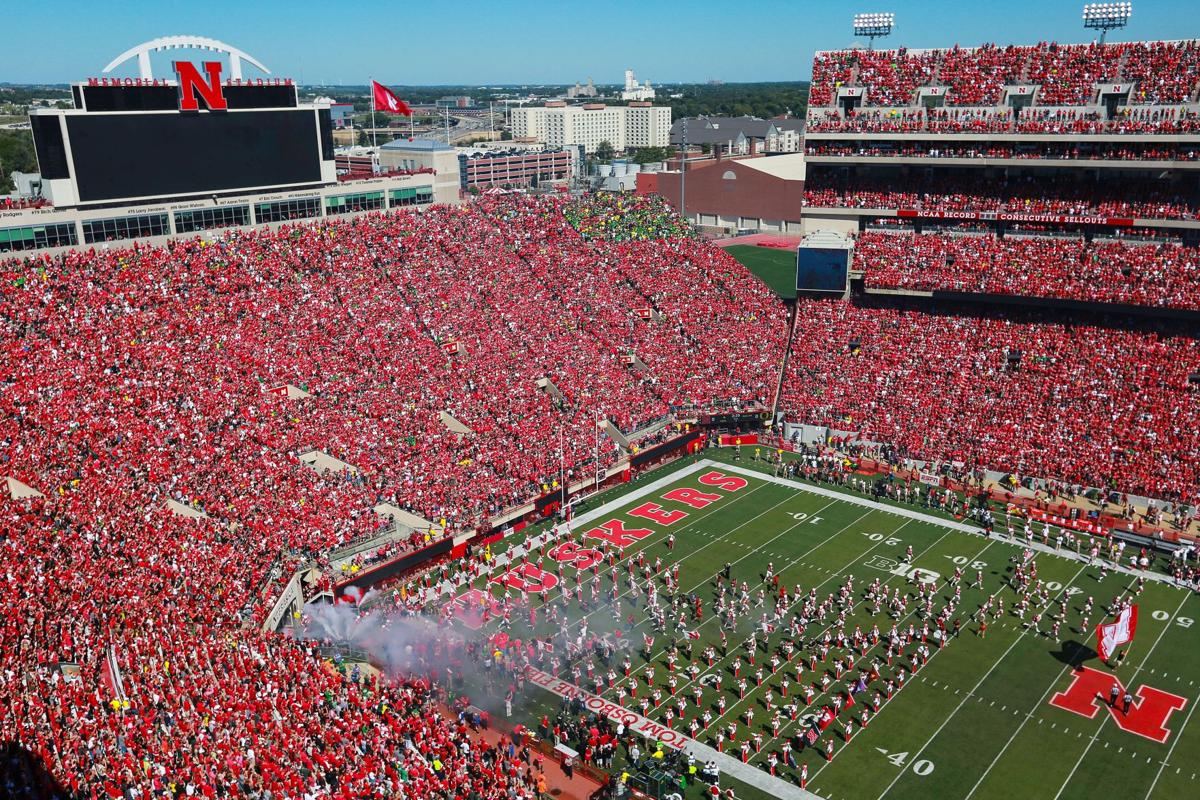This photo captures the vibrant atmosphere of a Nebraska Huskies college football game. The stadium, filled to capacity, creates a sea of red as enthusiastic fans clad in the team’s colors fill every seat in the sweeping bleachers that rise to the top. The field features a bright green expanse with a bold red "N" for Nebraska at the 50-yard line and "Huskies" prominently displayed in the end zone. The marching band, mid-performance near the end zone, adds to the lively scene as a flag-bearer proudly waves the Nebraska Huskies flag. A large black screen scoreboard, topped with a red "N," stands prominently on the left side. It is daytime, and the cityscape is faintly visible beyond the stadium, adding to the overall grandeur of the moment.